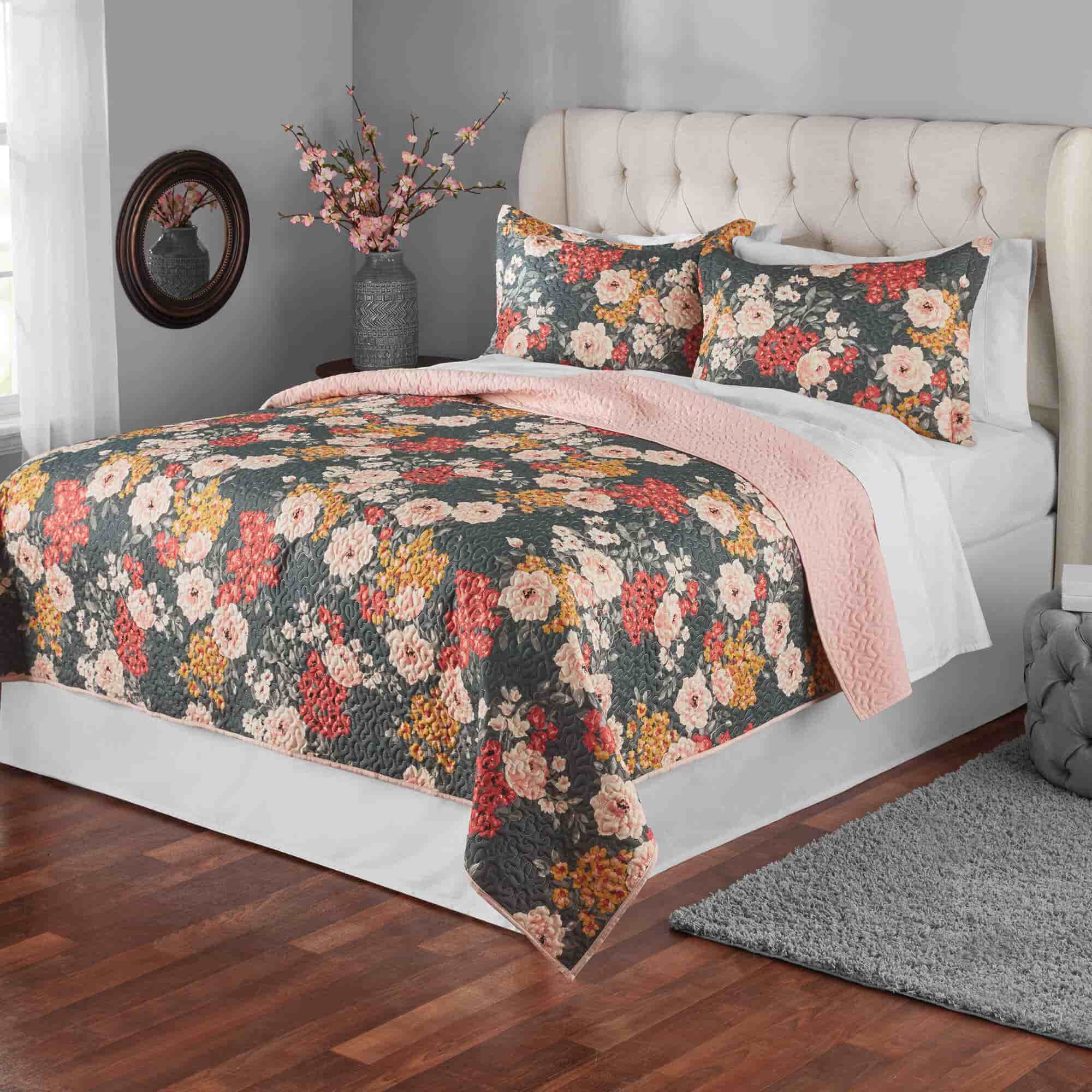The image showcases a meticulously organized bedroom featuring a large bed as its focal point. The bedspread sports a detailed floral design with white, yellow, and red flowers set against a grayish-green background. Complementing this are two pillows with the same floral pattern and two additional white pillows behind them. A portion of the blanket is folded over, revealing a pink underside. The bed has a cushioned white headboard and rests on a wooden floor with a gray throw rug to its right.

To the left of the bed stands a wooden nightstand holding a gray vase filled with pink flowers. Adjacent to the vase is a circular mirror with a brown border that reflects the flowers. The white walls and the edge of a window with white curtains further brighten the room, enhancing the overall sense of cleanliness and organization. The predominant colors in the room are white and various floral hues, creating a fresh and inviting atmosphere.